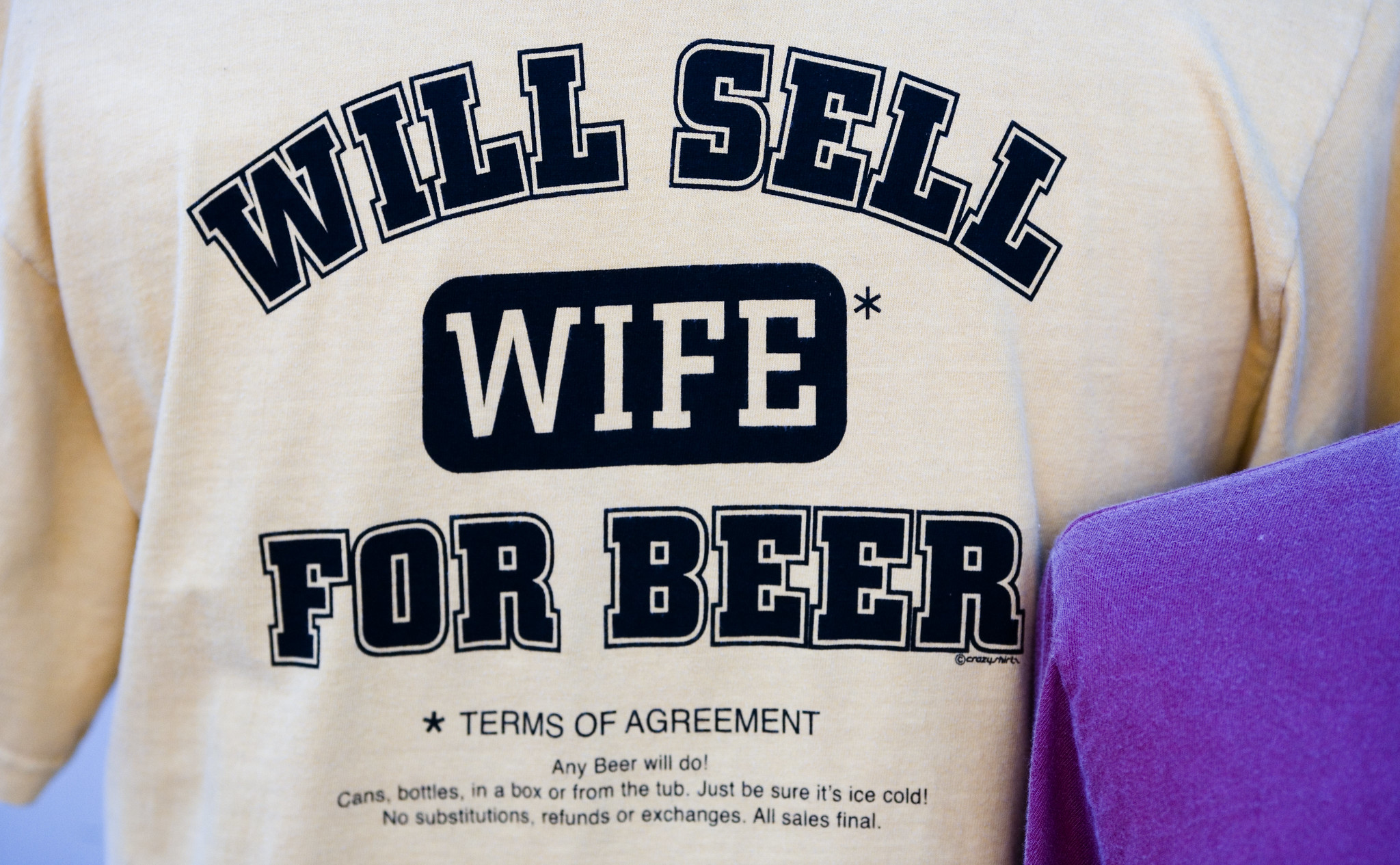This image features a short-sleeve white t-shirt with black lettering. The t-shirt's chest area displays the humorous message: "Will sell wife for beer." This text is arranged with "Will sell" curved at the top, "wife" prominently centered within a black rectangle, followed by "for beer" underneath. Beside the word "wife" is an asterisk that leads to smaller print at the bottom reading: "Terms of agreement: Any beer will do, cans, bottles, in a box or from the tub, just be sure it's ice-cold. No substitutions, refunds, or exchanges. All sales final." The scene includes a small section of purple fabric at the bottom right, likely another shirt, draped nearby. The background consists of white walls, highlighting the t-shirt as the focal point.